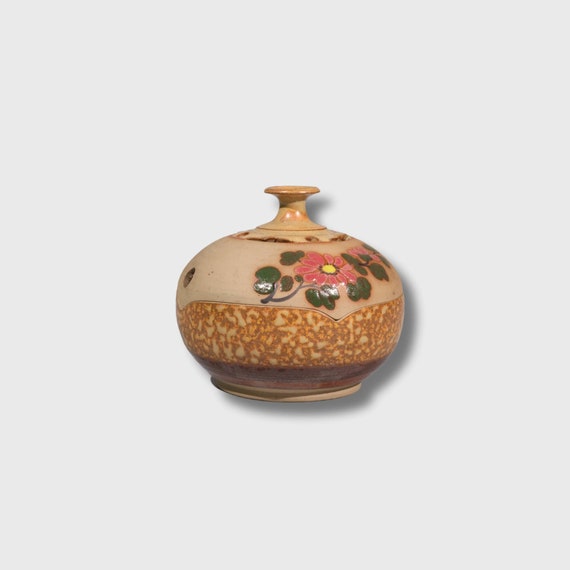This image depicts a handmade ceramic censer characterized by a bulbous, round body and a small opening at the top. The censer features a beige background that serves as the canvas for intricate floral designs. The bottom half of the censer showcases a modeled design with a beige background and an orange overlay, followed by bands of light and dark brown. Above these bands, a repeating pattern enhances its aesthetic appeal. 

The top half of the censer highlights a delicately painted pink daisy, complete with green stems and leaves, and a yellow center, adding a touch of natural beauty. The very top of the censer features a narrow neck that curves outward to form the small opening. This unique vessel, photographed against a light background, combines traditional craftsmanship with artistic floral detailing, making it both functional and decorative.